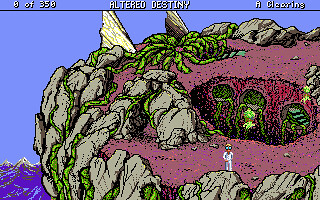A screenshot from the game "Altered Destiny" showcases highly detailed, vintage graphics reminiscent of early Windows or DOS systems. The image features a rugged cliff adorned with numerous rocks and vibrant plant life, set against a backdrop of majestic mountains under a bright blue sky. A character stands near the bottom right of the image, slightly off-center. The scene is suffused with a palette of dusty pinks, green chartreuse, yellows, and blues. In the upper part of the screen, the game's title "Altered Destiny" is prominently displayed, accompanied by a score indicator on the left which reads "0 of 350 points," suggesting a point-based mechanic for tracking progress. The right side of the screen includes text that describes the scene as "a clearing."